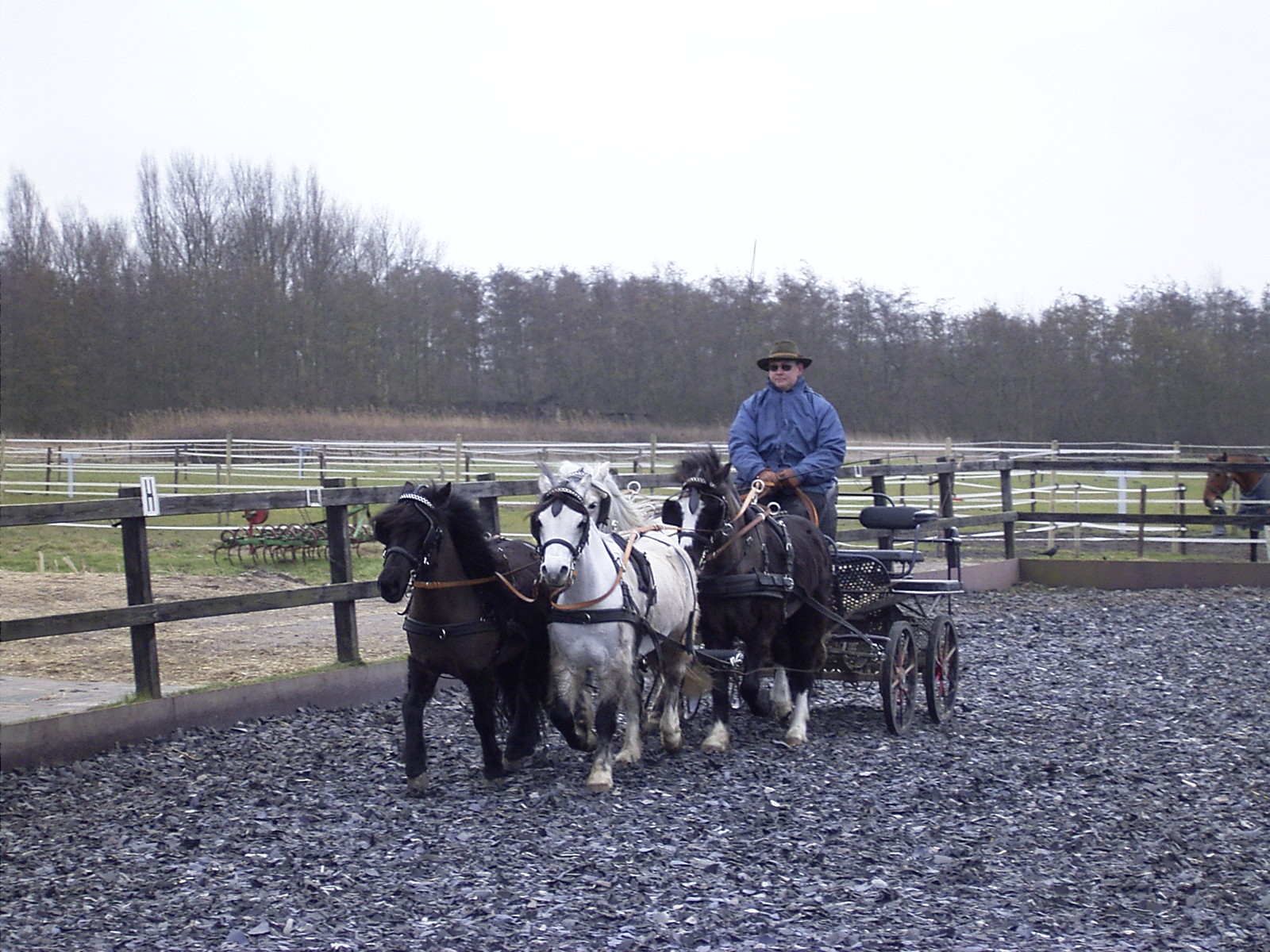In this vivid outdoor scene, a middle-aged man rides in an open, black, four-wheeled carriage, which is being pulled by a team of four small horses that resemble ponies. The man is dressed for cooler weather, wearing a blue raincoat, a hat, brown gloves, and sunglasses. The carriage moves across a surface covered in gray wood chips, within an enclosed farmyard or ranch area, fenced with a mix of white and brown barriers. The background reveals additional enclosures with at least one more horse visible. The surroundings also feature a line of leafless trees under a brightly lit, gray sky, indicating a chilly day in the countryside. The horses pulling the carriage are varied in color - black, white, and a combination of black and white - each harnessed and working as a coordinated team. This rustic setting suggests a peaceful yet active day on the farm.